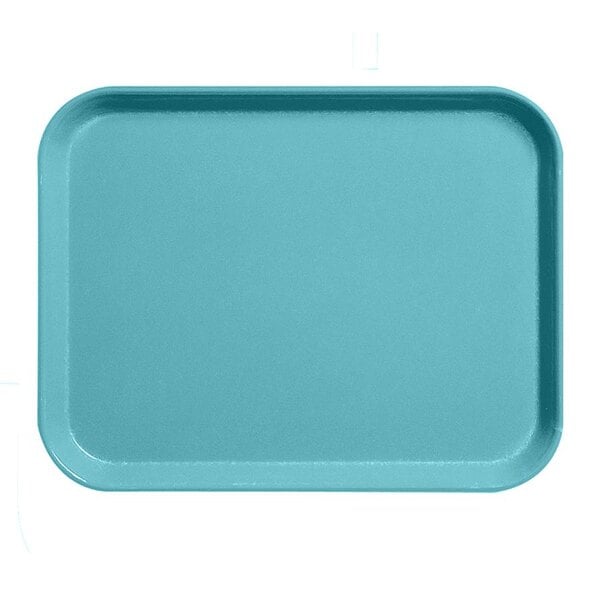The image features a singular, rectangular plastic tray with rounded edges, set against a completely white background devoid of any shadows or text. The tray is teal, exhibiting a bluish-green hue akin to sea foam, and appears to be standing upright. Due to the light source positioned at the top right corner, the left side and bottom of the tray are illuminated, while the top and right sides are in shadow, with a noticeable glare at the bottom left corner. The light's reflection on the plastic surface enhances its turquoise color, providing a clear indication of the tray's material and texture. The tray stands alone with nothing on or around it, making it the sole focus of the image.